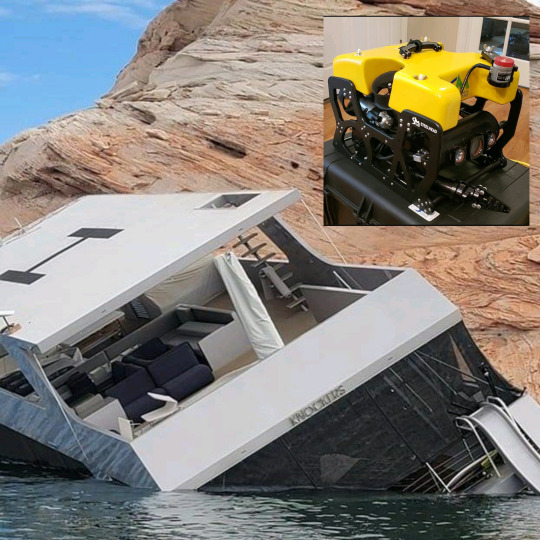The main photograph captures a dramatic scene set during the daytime, featuring a large, light-gray yacht labeled "Knockers" that has collided with a rocky cliffside and is in the process of sinking into dark green water. The yacht, tilted to its left, displays at least two or three layers, including an H-marked helipad on its top and children’s slides extending from its rear. The background showcases striking red and tan rock formations rising against a clear blue sky. In the upper right corner of the main image, an inset square image highlights a black and yellow motor, possibly an underwater diving robot, resting atop a black toolbox. This motor is situated on a wooden floor, bordered by a light wall and part of a doorway, suggesting an indoor setting.